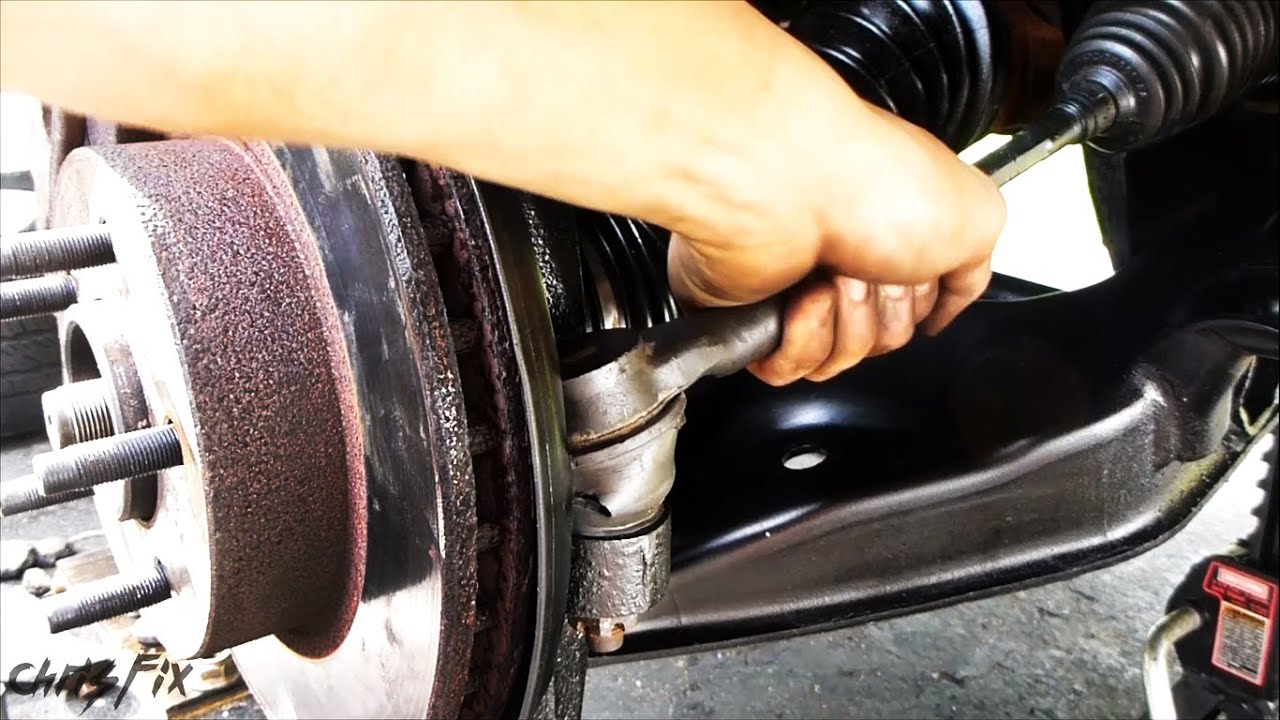This detailed artistic photograph, signed by the photographer Chris Fix in a slanted, handwritten style, captures a close-up scene of a mechanic's hand working within the intricate components of a car engine. The image prominently features a hand grasping a small bar inside the engine, with emphasis on various mechanical parts. An axle with protruding screws and a rusted rotor are visible, suggesting the tire has been removed and the vehicle is elevated. The mechanic’s white forearm hints at the hands-on adjustments being made, possibly to a strut that steers the wheel. The signature "Chris Fix," with its capitalized initials, appears in the bottom left corner, lending an artistic or promotional aspect to the photograph.